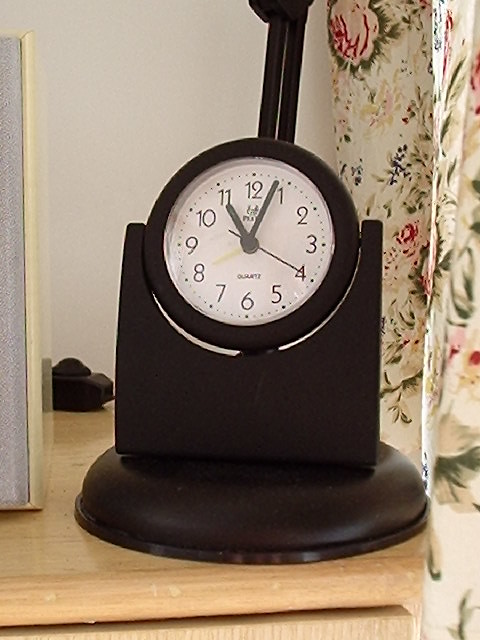This is an image of a tabletop clock placed on a light-colored wooden table. The clock features a rounded base that smoothly transitions into its circular casing, which is entirely black. The clock is held within a sleek, black holder with attachment points positioned at the 3 o'clock and 9 o'clock marks, suggesting a minimalist design. The clock face appears to be able to flip over, indicating that the reverse side may function as a mirror or serve another purpose. In the background, floral drapes with a cream-colored base are visible, adorned with intricate patterns of pink and reddish roses, green leaves, and yellow flowers. The wall behind the drapes is white, providing a clean and neutral backdrop to the scene.